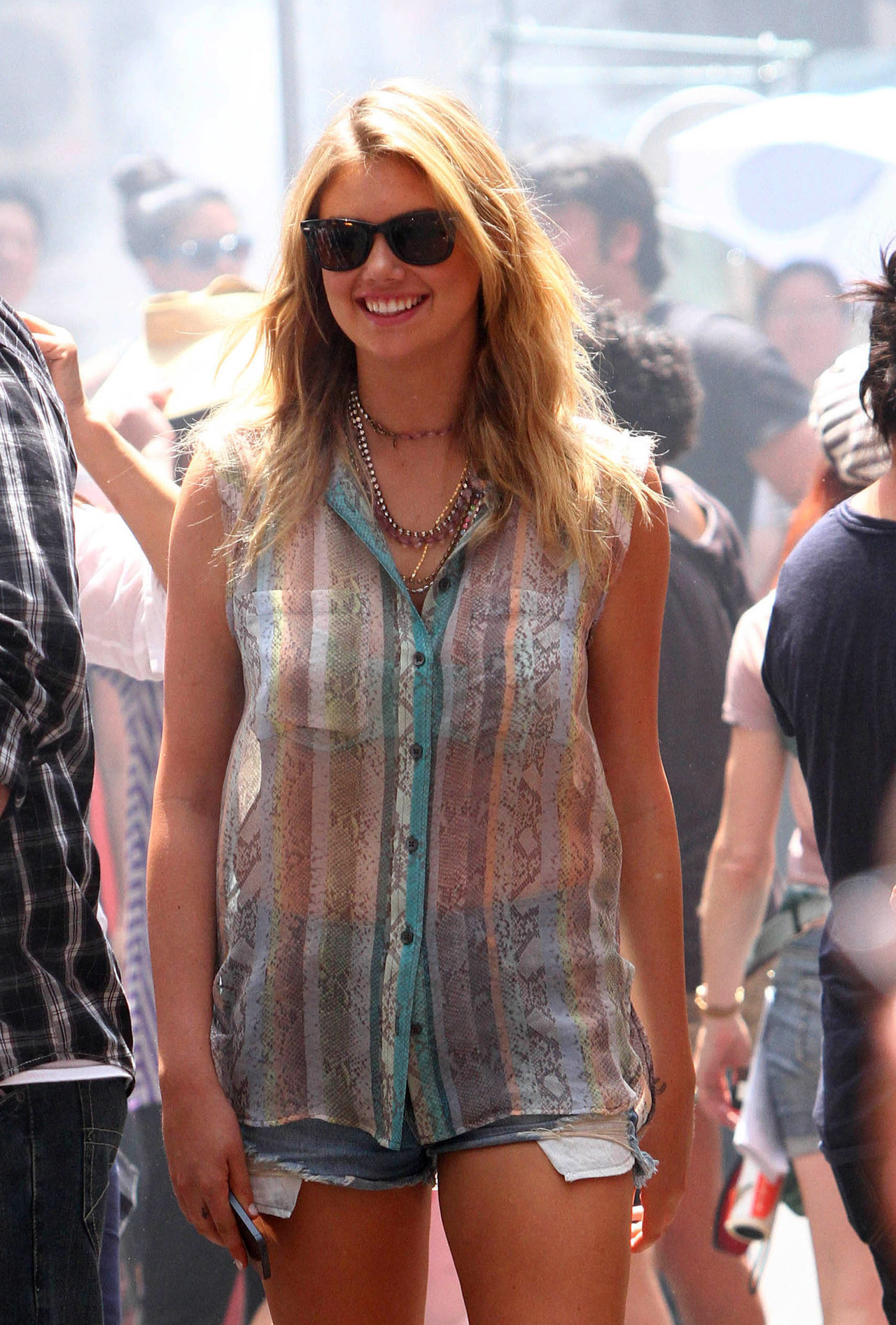The image features a young, attractive blonde woman, likely in her twenties, standing front and center amidst a large, bustling crowd. The background is slightly out of focus, filled with people walking around, suggesting either a busy street or an event. The woman is the main focus of the photo and is moving in the direction of the camera. 

She has long blonde hair flowing slightly past her shoulders and is wearing large, black sunglasses that cover much of her face. Her attire includes a distinctive, sheer, multicolored sleeveless top with abstract shapes and various stripes in pink, green, blue, orange, and yellow, under which she wears a white tube top. Completing her outfit are very short jean shorts with visible pockets that peek out from beneath the hem. 

Her accessories include several necklaces adorned with crystals and small circular gems. The woman is also smiling brightly, exuding a sense of joy and confidence. To her right, a person is wearing a black and white shirt, while to her left, another individual is seen in a dark sweatshirt. The crowd behind her, though blurred, adds to the sense of a lively environment. The overall scene is vibrant with colors like orange, teal, blue, and green, and there is also a hint of smoke in the background.